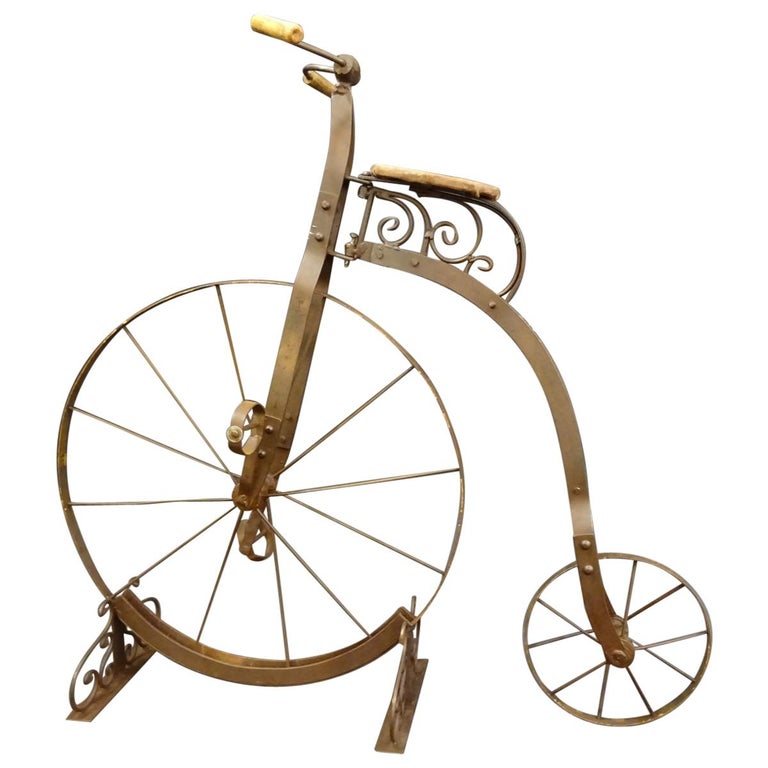This is a photograph of a tarnished gold metal bicycle sculpture, set against a white background. The vintage piece features one large wheel in the front and a smaller secondary wheel at the back. The handlebars have yellow or beige plastic grips, and the thin seat might be made of a different material, possibly plastic. The sculpture has intricate details like visible nails or screws, a filigree design around the seat, and it rests balanced on a metal stand made of the same gold material. The pedals are positioned in such a way that they appear to clip through the large front wheel, emphasizing the stationary nature of the piece. The overall design is evocative of an old-time high-rise bicycle, giving it an ornate, antique appearance.